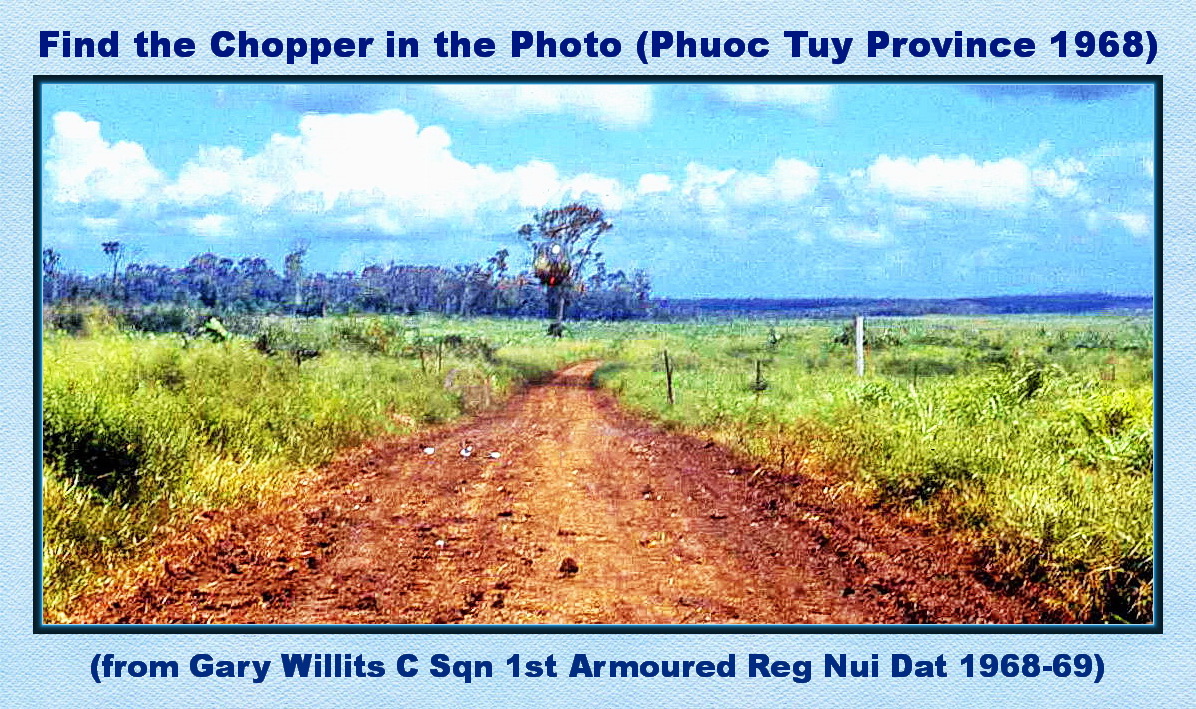The photograph, encased in a dark navy pinstripe border with a thicker light blue frame, invites viewers to "find the chopper in the photo" with additional text indicating the location "Phuoc Thuy province, 1968". Beneath the image, the caption reads, "from Gary Willett, CSQN, First Armored Reg., Nui Dat, 1969". Set in a landscape orientation, the image presents a vibrant scene with a blue sky dotted with white clouds and a purplish-blue horizon. In the foreground lies a reddish-beige and brown dirt road that narrows as it recedes into the distance, flanked by tall, green, and yellow grasses and plants. Centered above the horizon is a distinctive row of blue trees. Amidst these trees, partially concealed, is the elusive helicopter, identifiable by its shadow on the road. The helicopter is subtle, resembling a clear spherical shape with a blue fringe, a small red dot at the bottom, a white dot at the top, and a blurred, slanted propeller blade.